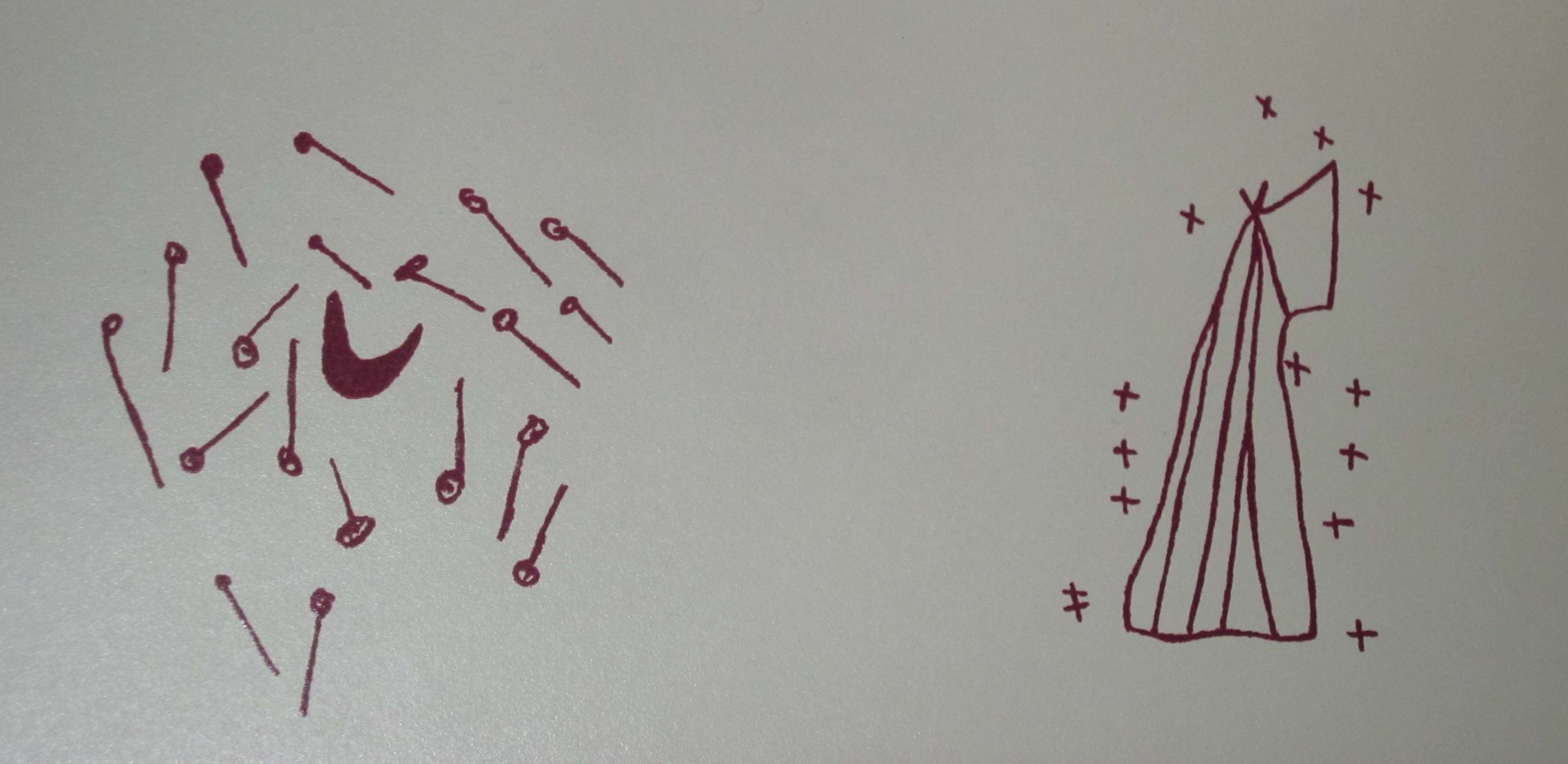The artwork is a drawing that combines elements reminiscent of ancient hieroglyphics or cave drawings with the precision of a modern diagram. Rendered in red, possibly maroon ink or marker, the left side features numerous pins arranged around an upward-facing crescent moon. To the right, an enigmatic structure resembling a teepee fused with a V shape emerges. This form includes protrusions akin to sticks, possibly symbolic rather than literal. The descending lines within the V evoke the texture of tree bark, and a small ax blade shape extends from the top, adding to the complexity of the design. Intriguingly, one might also interpret the shape as a seated dog gazing skyward. Surrounding this central motif are numerous crosses, akin to tiny stars, suggesting an astrological theme. The precise meaning remains elusive without additional context, but the drawing clearly strives to convey a celestial or symbolic narrative.